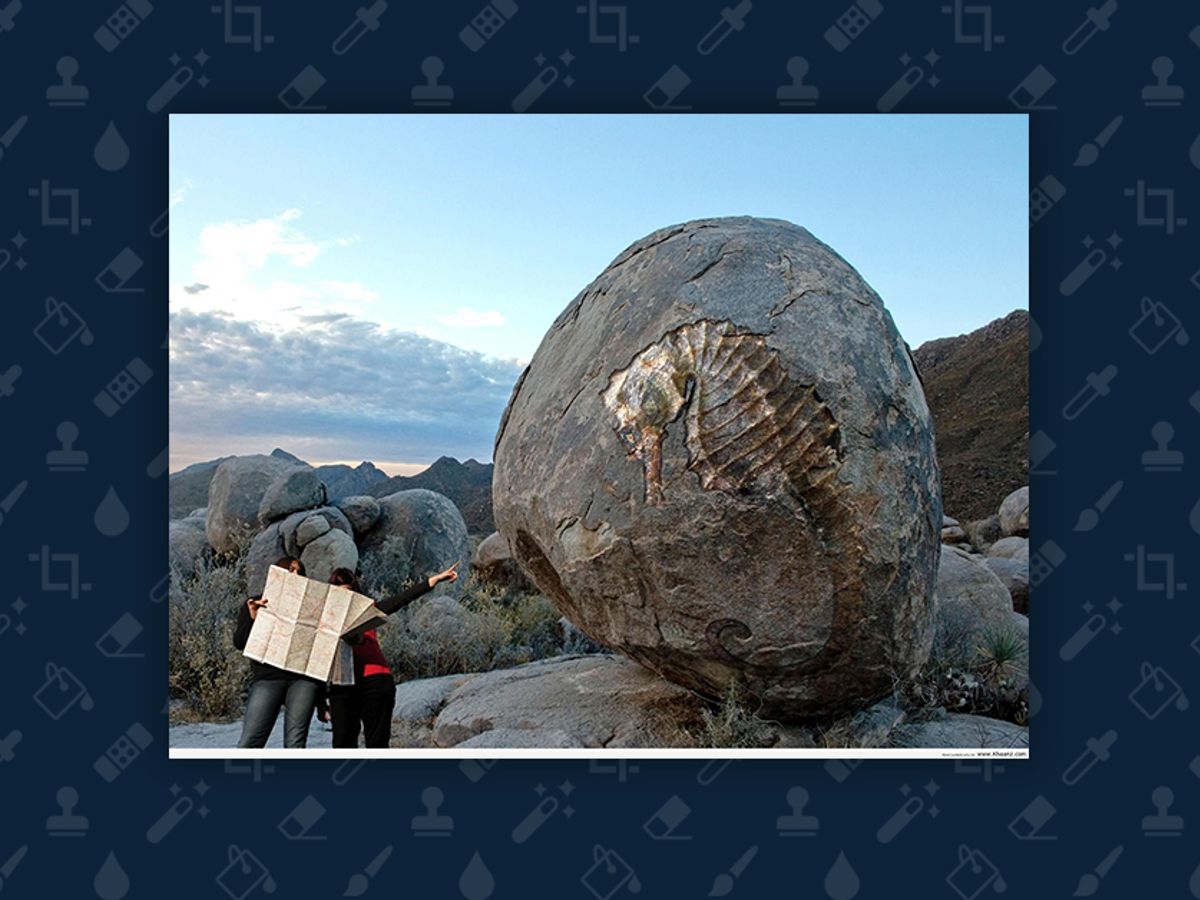In this vivid outdoor photograph, two tourists with long black hair stand in a rugged mountain area, the sky above them a bright blue adorned with low clouds. They are engrossed in examining a map, one of them wearing a red long-sleeve shirt with black pants, and the other dressed in a black shirt paired with blue jeans. The focus of their attention—and the image—is a colossal, roughly circular rock that towers three times their height and is about five times their width. Carved into its side is a striking golden coppery seahorse, which stands out against the natural rocky landscape. This monumental stone may also have an opening in its center. The scene includes a backdrop of additional rocks and hills, enhancing the sense of grandeur. The photograph, bordered with dark blue icons such as a stamp, eraser, paint bucket, ink dropper, magic wand, water droplet, and squares, adds an artistic touch to the overall presentation.